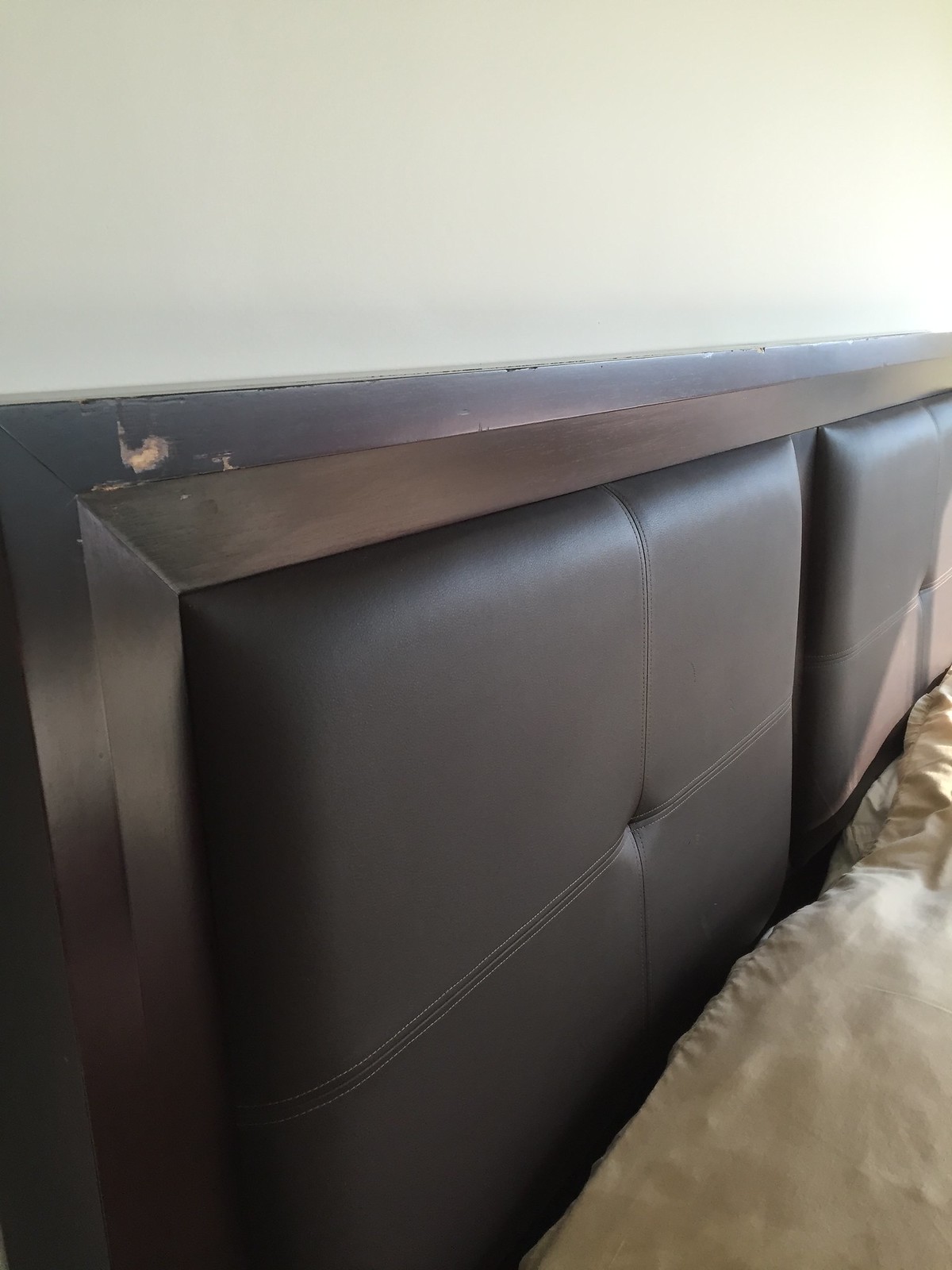The photograph, taken from a diagonal angle on the left side of the bed, captures a partial, close-up view of a dark-stained wooden headboard against a white wall. The headboard features a prominent chip in the upper left corner, revealing a lighter wood beneath the dark stain. The headboard has an angled, triangular shape at the top and is marred with additional scuffs and dinges. It includes a padded brown leather section designed like a headrest, consisting of four individually sewn panels with a central button. At the bottom right of the image, a yellowish or light gold-colored, silky blanket is pulled up to the headboard. The headboard is positioned against a cream-colored wall, creating a contrasting backdrop for the scene.